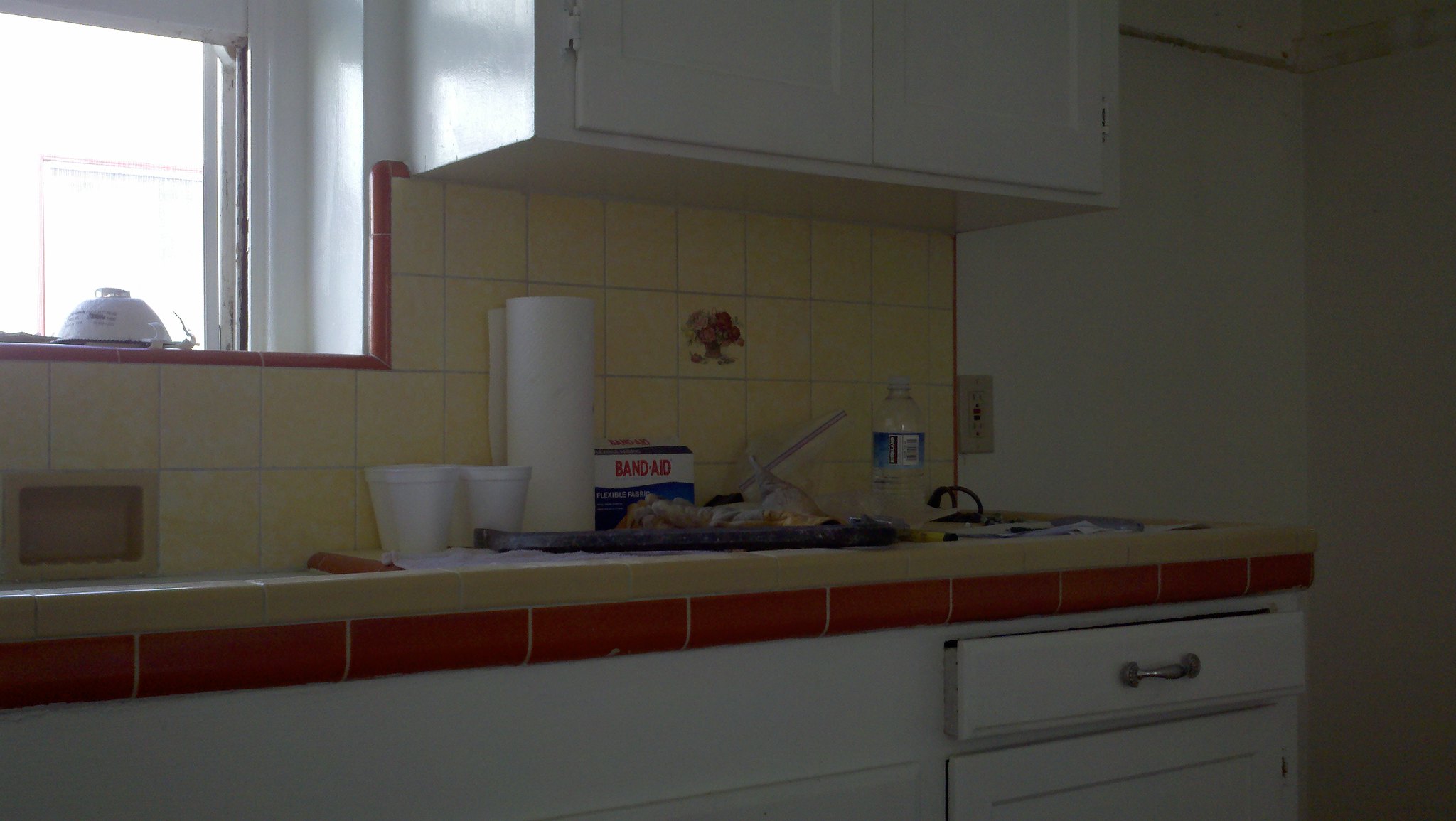A photo of a kitchen countertop is presented, taken from a perspective that angles slightly to the right, offering a straight-on view. To the left, above the countertop, a window allows natural light to pour into the space. This window sits directly above the sink. Adjacent to the window is a white cabinet that adds a touch of brightness to the setup. The countertop itself is a warm tan color, creating a harmonious contrast with a line of reddish terracotta brick-inspired tiling that runs just below its edge. Above the sink and beneath the countertop, the backsplash area features a blend of tan and white marble-like tiles, trimmed neatly with the same terracotta brick-style edging. Outside the window, sunlight can be seen reflecting off surfaces, casting a gentle glow into the kitchen. A partially opened drawer with a sleek silver handle is also visible, along with a light switch or electrical outlet located on the left side of the scene, completing this detailed kitchen vignette.